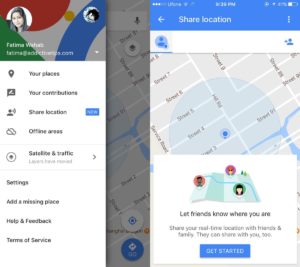In the screenshot provided, we observe a very small and blurry image, presenting a variety of elements that give us an overall impression of the interface. At the top, there is an arrow pointing to the left next to a 'Share Location' indication. On the left side of the screen, there is a small circular avatar featuring an individual named Fatima, who is smiling in the photo.

The top portion of the screen has a blue background and includes subtle interface elements such as a battery indicator, three dots menu, and the current time, which are barely visible due to the image's small size. 

Following this, a menu bar is visible listing several options such as 'Your Places,' 'Your Contributions,' 'Share Location,' 'Offline Areas,' 'Satellite,' and 'Traffic,' each accompanied by right arrows. Additional options include 'Settings,' 'Add a Missing Place,' 'Help and Feedback,' and 'Terms of Service.'

In the middle of the screen's right portion, there is a map image illustrating Fatima's location, highlighting the app's real-time location-sharing feature. The bottom of the screen features a 'Get Started' button, encouraging users to initiate the location-sharing process.

Overall, this is a screenshot depicting the location-sharing interface for an individual named Fatima, providing options for users to share their real-time location with friends and family.